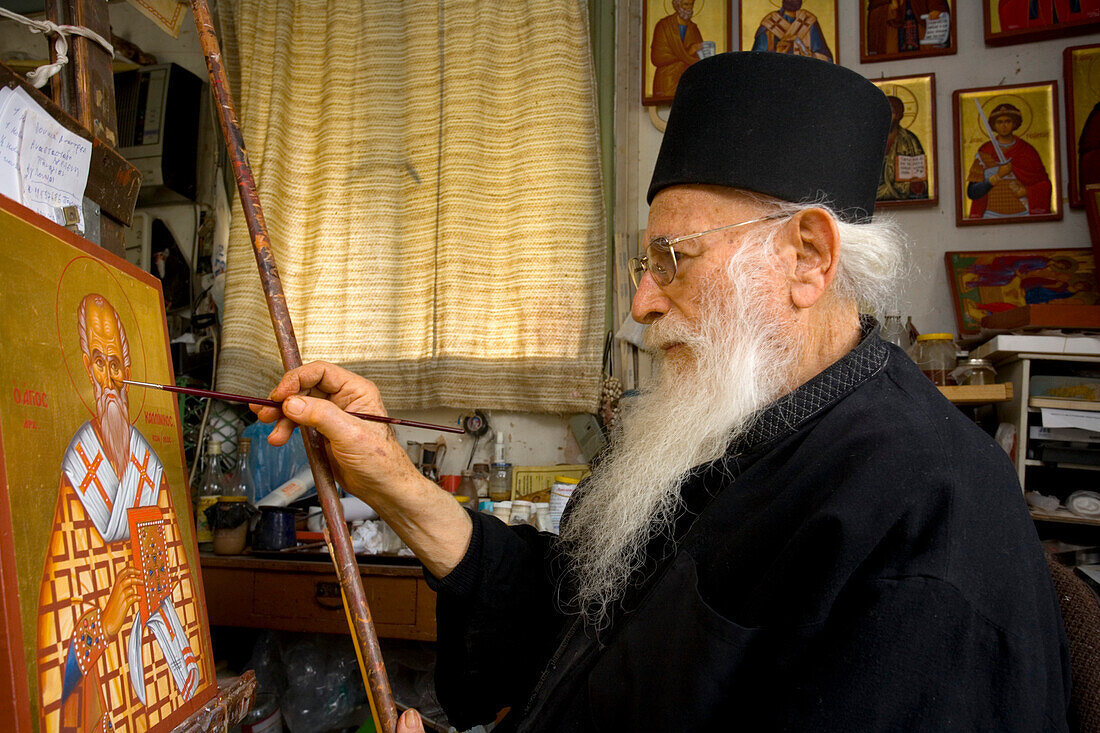The photograph captures an elderly man, likely a painter, engrossed in his craft. The man, visible from the waist up, sports a long white beard and mustache, metal-framed glasses, and a distinctive black round cap. His black robe, with its sleeves pulled back to his mid-forearms, suggests he is deep into the process of painting. He is painting a detailed portrait on a rectangular canvas positioned on an easel. The painting features a bearded figure in white and yellow robes adorned with crosses, a halo behind his head, and a book in his hand, possibly an apostle. The background of the canvas is a rich gold.

The painter uses a large wooden stick to steady his hand as he works with a red paintbrush. Behind him, a white wall is adorned with multiple framed religious icons and paintings, contributing to the room's devotional ambiance. To his left, light filters through a window covered by a striped, slightly dirty curtain. Surrounding the painter are a variety of painting supplies and equipment, scattered across a dark wooden desk, adding a touch of organized chaos to his creative space. Overall, the image captures a serene, detailed moment of artistic creation steeped in religious iconography.